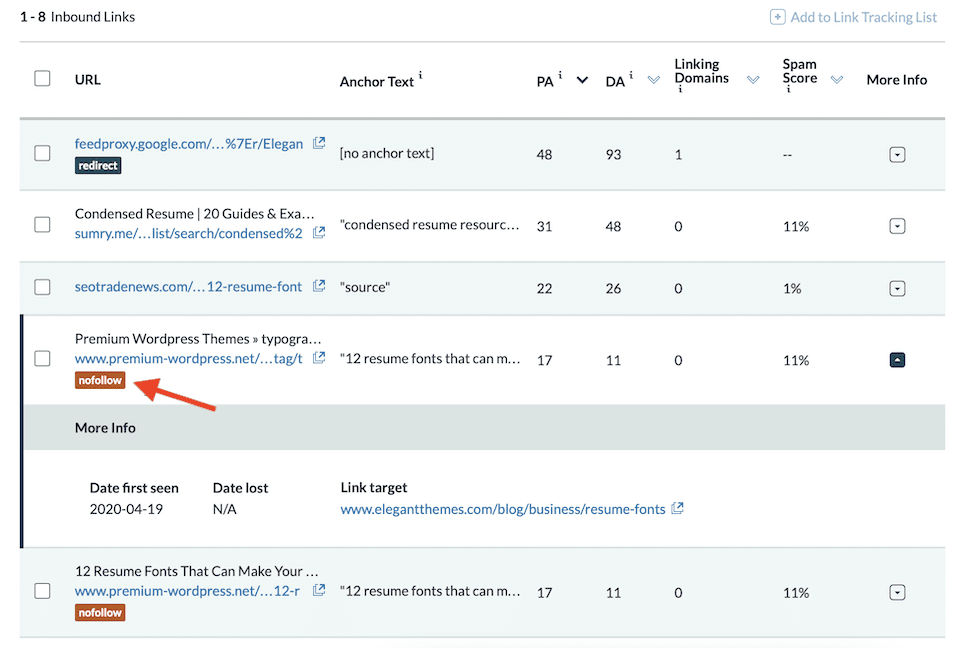This image showcases a web interface from an SEO tool designed to track, analyze, and manage inbound links. The interface provides comprehensive details for each link, including the URL, anchor text used, page authority (a metric that indicates the authority of the page), domain authority, linking domains, and spam score. 

In the list:
1. The first entry is from feedproxy.google.com, but the link appears to be broken.
2. The second entry is also a broken link.
3. There are six links in total on display, with one discernible link possibly from elegantthemes.com, which hosts a blog.
4. Another entry appears to be from a WordPress site.

The interface allows users to check a box next to each link to add it to a tracking list, and certain entries can be expanded for more detailed information. This tool is pivotal in evaluating the quality and relevance of inbound links through various metrics and insights.